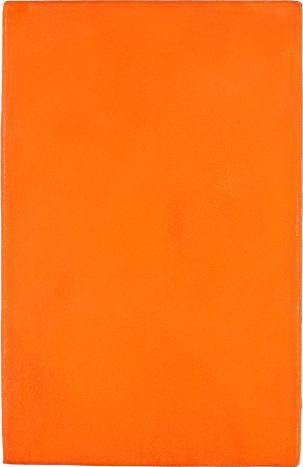The image depicts a solid orange rectangle, reminiscent of a book cover or a door, with a burnt orange hue that strikes a balance between boldness and subtlety. The rectangle is oriented vertically, being taller than it is wide, much like a portrait. The corners and sides of the rectangle are slightly worn and not perfectly straight, showing minor curvature and imperfections, which adds a touch of character. A faint line of discoloration is visible on the left side, while there's a subtle wear line running down the far right side. Set against a plain white background, the rectangle stands out as a solitary, vibrant object, exuding a warm yet minimalistic aesthetic.